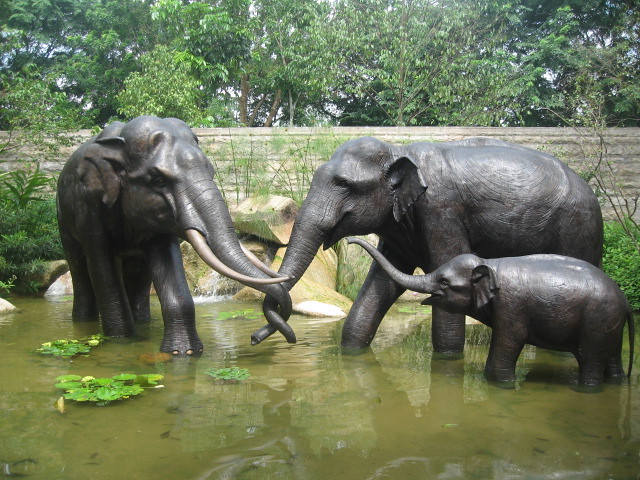This photograph captures an outdoor art installation featuring lifelike statues of three elephants standing in a shallow pond. Prominently situated are two large elephants and a smaller one, signifying a family unit. The larger elephant on the left boasts long tusks, marking it as the male, while the slightly smaller female on the right lacks tusks. Their trunks tenderly intertwined suggest a gesture of affection. Nestled closely, the baby elephant stands beside the female, trunk joyfully raised as if relishing the familial bond. The pond, murky and adorned with clusters of green lily pads, envelops the elephants' feet. The scene is enriched with natural elements, including scattered rocks, bushes, and reeds emerging from the water. In the background, a substantial concrete wall borders the installation, beyond which various trees stand tall, providing a lush, natural backdrop to this serene family tableau.